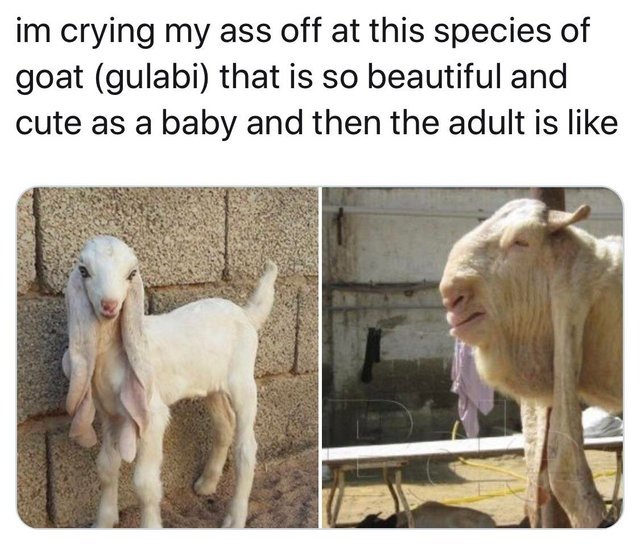This image showcases a striking contrast between two Gulabi goats, highlighting the stark difference in appearance as they age. On the left, a charming baby goat stands beside a concrete wall, entirely white and fluffy with extraordinarily long ears. Its cute little face, adorned with a tiny nose and expressive eyes, makes it utterly adorable. The setting includes some cinder blocks or big brick in the background and it appears to stand on sand or bedding. In contrast, the right side of the image features an adult Gulabi goat, which appears rather startling. The adult's face is marked by saggy skin that nearly obscures its eyes, and its long ears have transformed into what looks like hanging extra skin. The older goat's head is visible against an outdoor backdrop filled with old buildings and scattered boards. The caption humorously underscores this dramatic transformation, reading, "I'm crying my ass off at this species of goat, a Gulabi, that is so beautiful and cute as a baby and then the adult is like..."